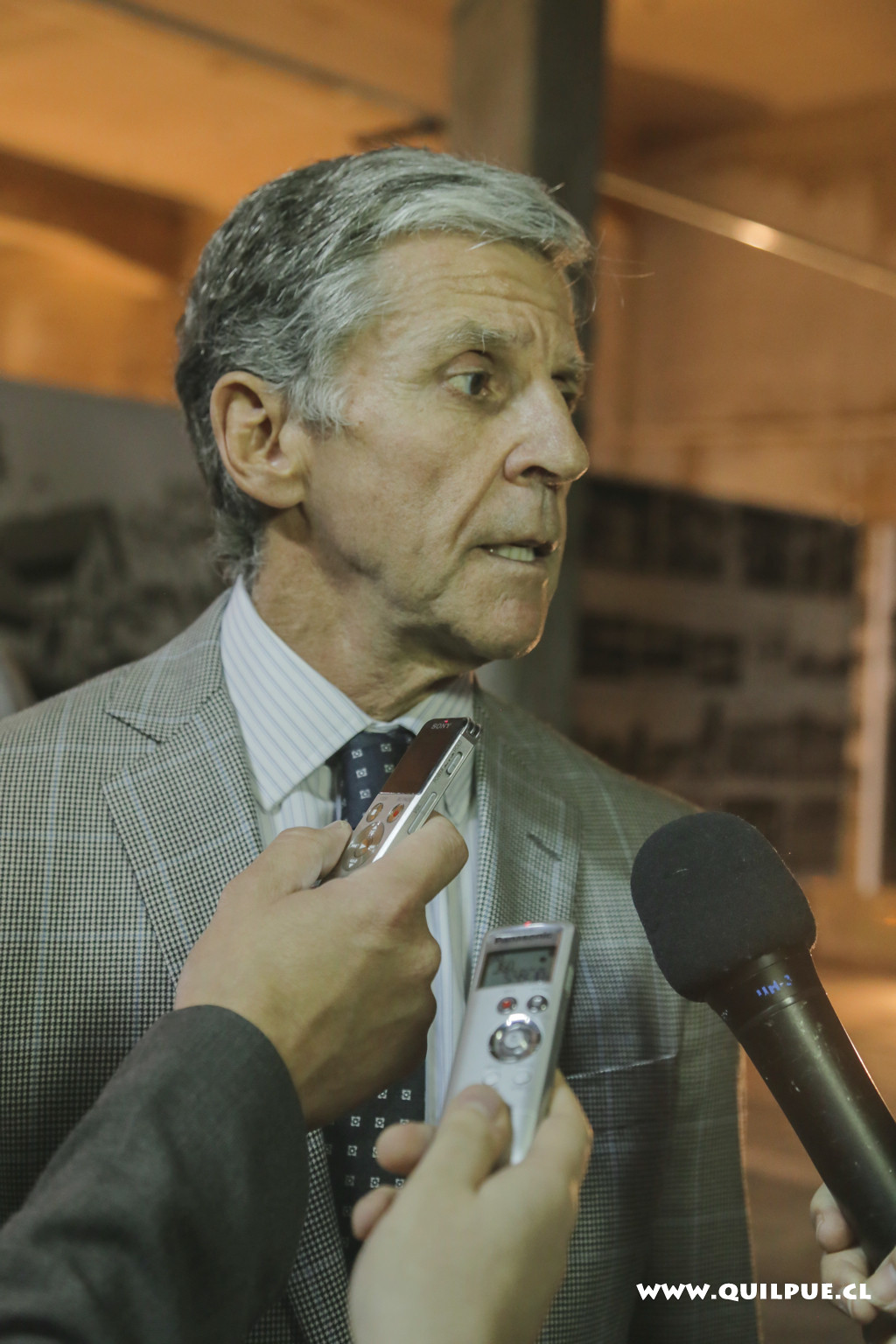In the center of the image stands an older man with salt and pepper hair, predominantly gray. He has an olive complexion and is dressed in a gray flannel suit with a checkered pattern, complemented by a white and blue striped shirt and a navy blue tie. The man, positioned directly in the middle of the frame, is glancing to his left, towards the right side of the image. He appears to be in the midst of an interview, surrounded by multiple journalists. Three hands are visible, each holding a different recording device: the left hand, clad in a dark gray jacket, holds a silver recorder; the middle hand holds another silver recorder; and the right hand holds a black microphone. The backdrop of the image suggests an indoor setting, possibly resembling a street or parking garage, with a stone-like wall and some lighting. The website "www.quillpew.cl" is visible in white text at the bottom right corner of the image. The overall color palette includes shades of black, white, gray, tan, silver, and brown.